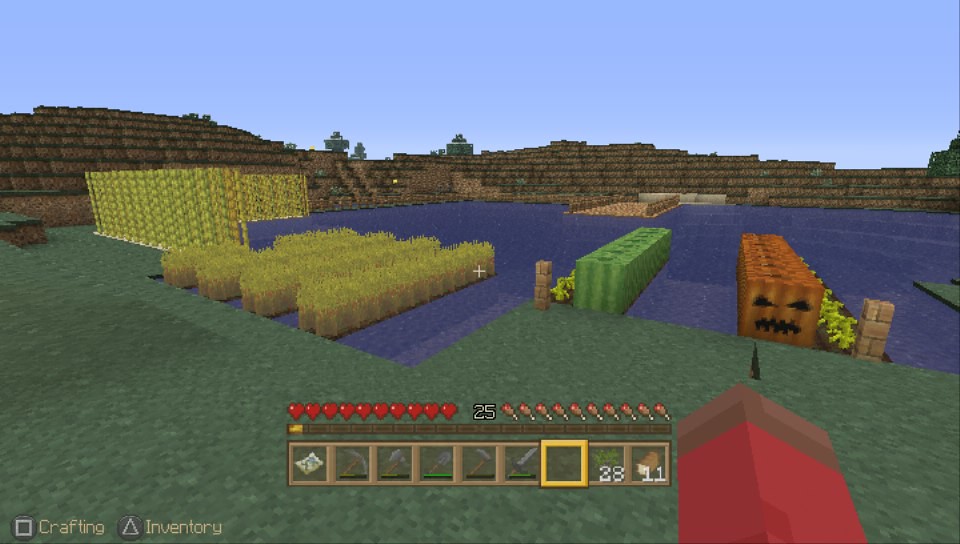The image is a detailed screen capture from a Minecraft-like video game with pixelated, retro-style graphics set in a vibrant and varied landscape. In the foreground, there's a vivid depiction of a blue-tinted lake or unusually colored grass, juxtaposed with patches of green and orange, the latter resembling pumpkin faces. Scattered bales of yellow hay contribute to a rustic atmosphere, some arranged to form low walls. The scene appears to be situated within a rocky canyon, its stone towers faintly visible in the background, adding a sense of depth and scale.

On the left side of the screen, there are user interface elements labeled "Crafting" and "Inventory," represented by square and triangular buttons. Additionally, a heads-up display (HUD) occupies another part of the screen, showcasing the player's vital statistics: hearts for health, turkey legs for hunger, a count of 25, pickaxes and other mining tools, 28 pieces of leavened bread, and a shrub-like item. The player's perspective is from the first-person view, with only a red appendage or weapon visible, emphasizing their direct interaction with the environment.